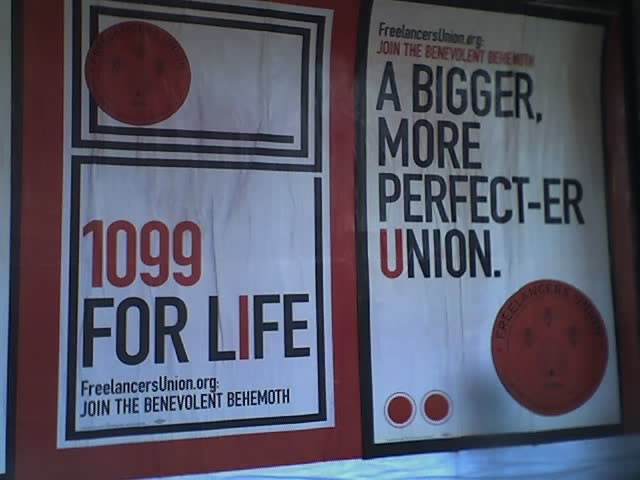This image captures two slightly crumpled posters displayed side by side on a red board, likely outdoors. The overall color scheme of the posters is a striking combination of red, black, and white, with large, bold text and geometric elements such as squares, borders, and circles. Both posters prominently feature the phrase "$10.99 for life, freelancersunion.org, join the benevolent behemoth." 

The poster on the right additionally reads "a bigger, more perfect-er union" in a larger, eye-catching font. Each poster is adorned with red emblems or seals, presumably the logo of the Freelancers Union, adding a formal touch. The dim lighting and the worn, textured surface of the posters suggest they've been exposed to the elements, possibly rain, before drying, giving them a rugged look.